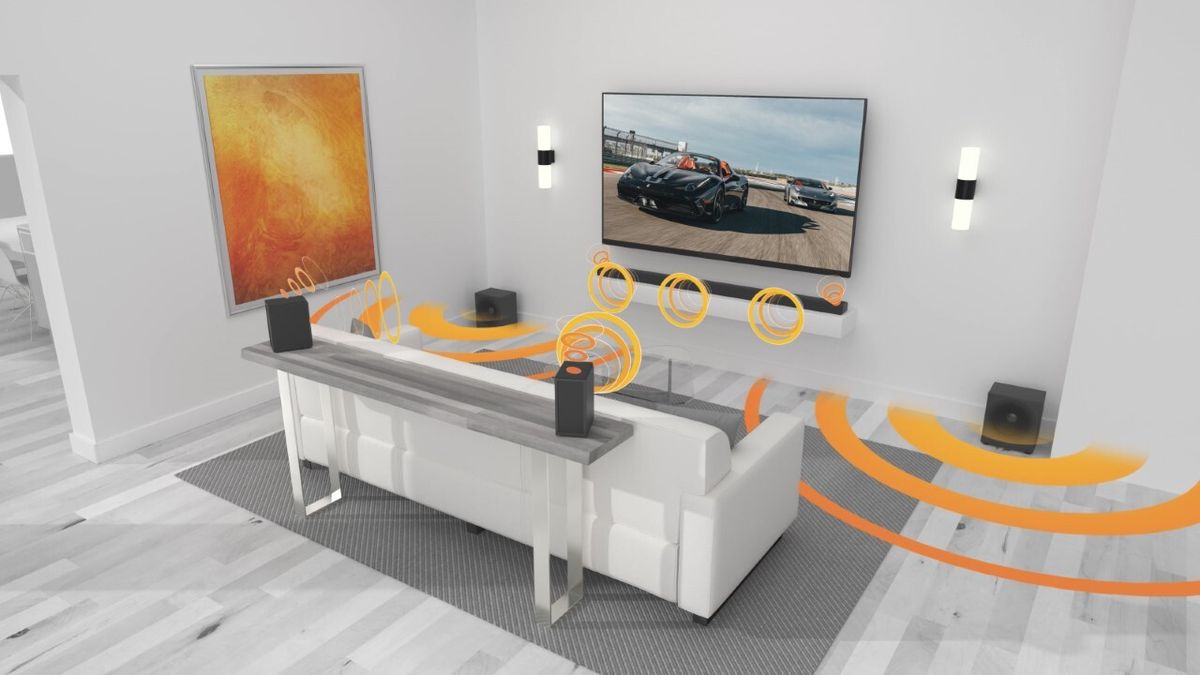The image is a high-definition, computer-generated illustration of a contemporary living room. Dominated by a sleek, white, modern-looking couch positioned directly in front of a large flat-screen TV mounted on the wall, the room is meticulously arranged to exude both comfort and high-tech sophistication. The TV screen depicts two race cars zooming past each other, delivering a sense of dynamic motion. Augmenting this high-tech setup is an elaborate surround sound system, visually represented by vibrant orange sound waves emanating from four strategically placed speakers – one in each corner of the room.

The room features a monochromatic color scheme with black and white furnishings, further accentuated by the stark contrast of the orange overlays used to illustrate the sound waves. The floor appears to be black and white hardwood, complementing the overall modern aesthetic. On one side of the room, a large, expensive-looking abstract painting in hues of orange and red adds a burst of color to the otherwise monochrome setting. Additionally, the wall houses two lights flanking the television and a soundboard situated beneath it, enhancing the immersive audio-visual experience for anyone seated on the couch.